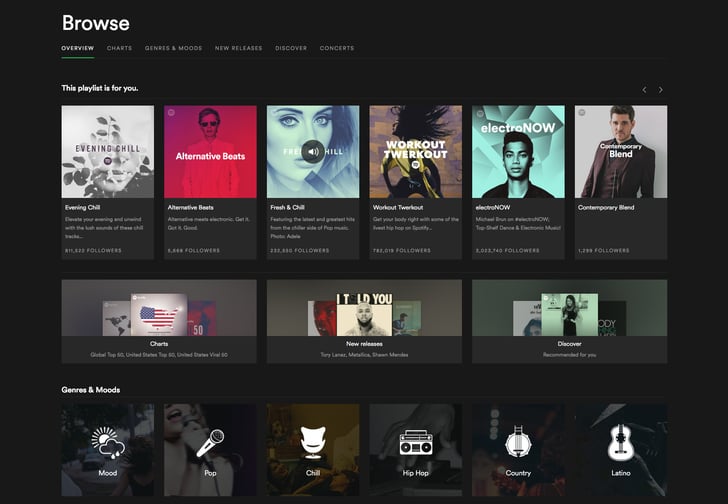Screenshot of the Spotify desktop app in dark mode. The user is browsing through the general music discovery area. The interface displays personalized playlists created for the user, with headings such as "This Playlist is For You," "Evening Chill," "Alternative Beats," "Fresh and Chill," "Workout Twerkout," "Electro Now," and "Contemporary Blend," indicating an advanced algorithm tailored to the user’s tastes based on their listening history. The sidebar offers quick access to curated sections like "Charts," "New Releases," and "Discover," as well as genre-specific categories including "Pop," "Chill," "Hip Hop," "Country," and "Latino." Tabs at the top mirror these categories, providing organized and streamlined navigation within the app.